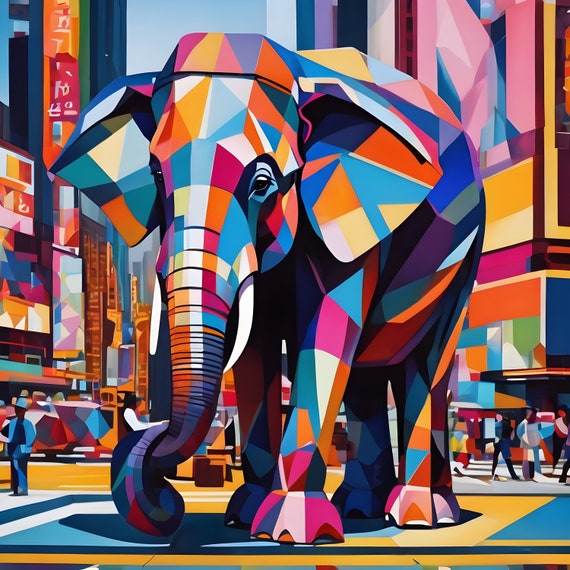The vibrant, comic book-style image features a colossal, geometrically constructed elephant standing prominently in the heart of Times Square. The elephant's form is an assemblage of rectangles, squares, and triangles, creating a captivating mosaic of colors, including vibrant shades of pink, orange, purple, blue, teal, yellow, and white. Its tusks are stark white, and its eyes are a striking pure black. Surrounding the elephant are the bustling pedestrian sidewalks and the busy streets filled with vehicles, all rendered in the same colorful geometric style. Behind the elephant, the iconic skyscrapers and billboards of Times Square loom, depicted with a similar array of multi-colored shapes and patterns. The scene is lively with people in the background, also stylized in geometric forms, adding to the dynamic and colorful urban backdrop. The elephant stands serenely amidst the chaos, a stunning blend of art and cityscape.